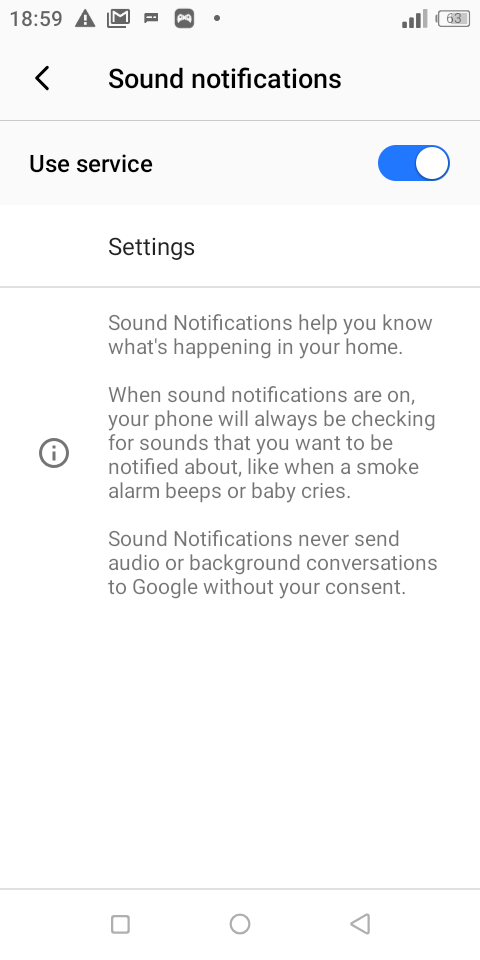Screenshot of an Android Device in Sound Notifications Settings

This detailed screenshot, likely captured from an Android phone, showcases a specific area within the device's settings. In the upper right-hand corner of the image, the status bar indicates a battery life at approximately 50%, alongside three bars of cell service signal but without a visible Wi-Fi icon. The time displayed is 18:59, and the notification area includes various icons such as Gmail notifications and an alert signified by an exclamation point within a triangle.

Central to the image is the "Sound Notifications" section within the settings. The header "Sound Notifications" is accompanied by a left-pointing arrow for navigation. Directly below, there is an option labeled "Use service" with a blue toggle switch indicating that the service is activated.

Further beneath, there is an informative paragraph outlining the function of sound notifications. It explains that these notifications assist users in staying aware of activities in their home, such as smoke alarms or a baby crying. It reassures users that sound notifications do not send any audio or background conversations to Google without permission.

The entire section is presented on a white background, and at the bottom of the screenshot, the typical Android navigation buttons are visible.